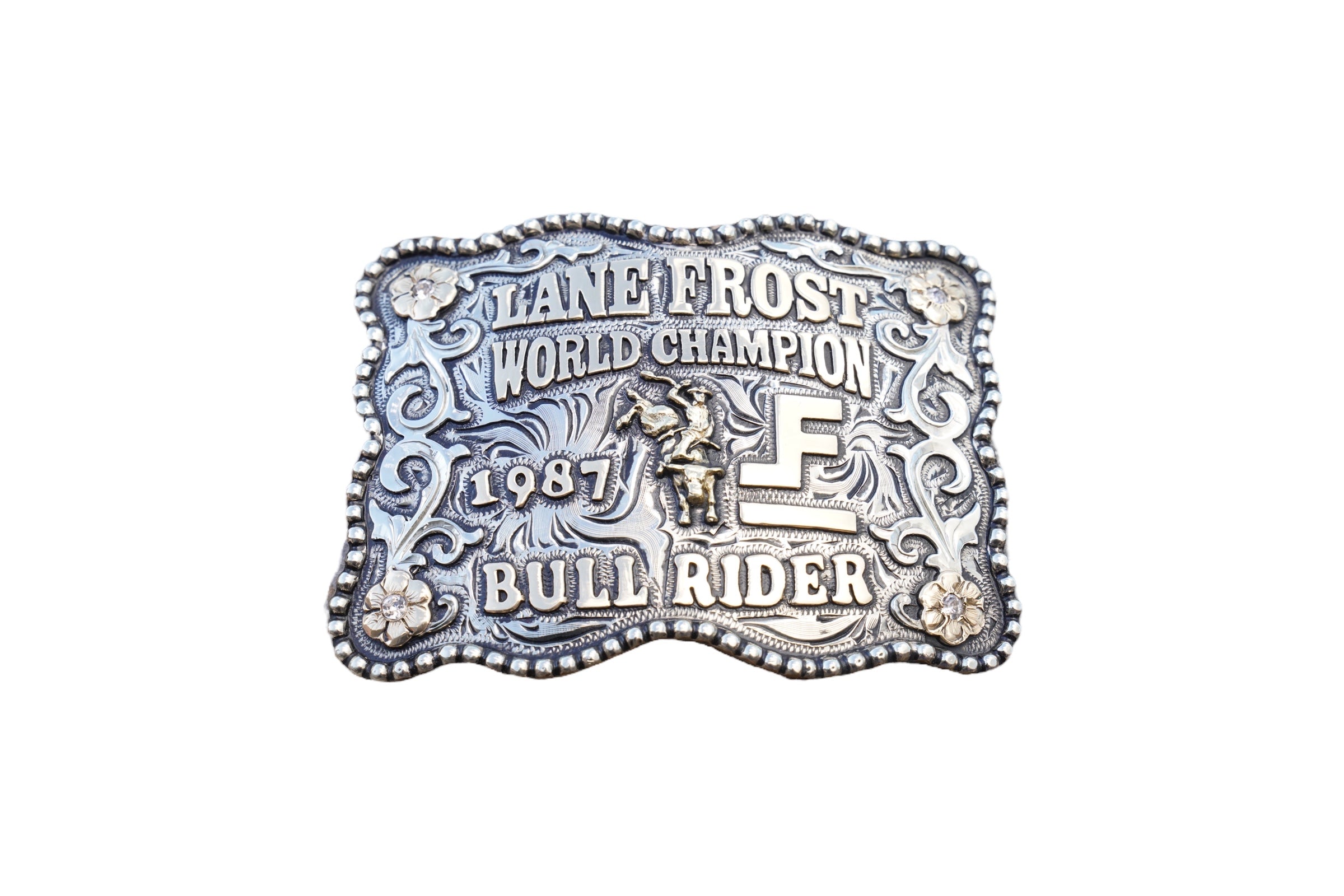This image depicts a commemorative silver belt buckle celebrating Lane Frost, the World Champion Bull Rider of 1987. The buckle features a highly detailed, ornate design. Along the outer edge, there is a beaded detail comprising small cylinders arranged sequentially, giving it a textured, curved outline. Inside this border, the main surface showcases an intricate flowery pattern, with each corner adorned by a flower and connected by leafy designs. The central focal point of the buckle includes a dynamic depiction of a man riding a bull, with the bull depicted in mid-kick, its back legs raised and the rider holding on with one arm. Above this image, the text reads "Lane Frost, World Champion," while below it, "Bull Rider" and the year "1987" are prominently displayed. The overall style and craftsmanship suggest this buckle serves as a prize or commemorative item from Lane Frost's championship victory in 1987.